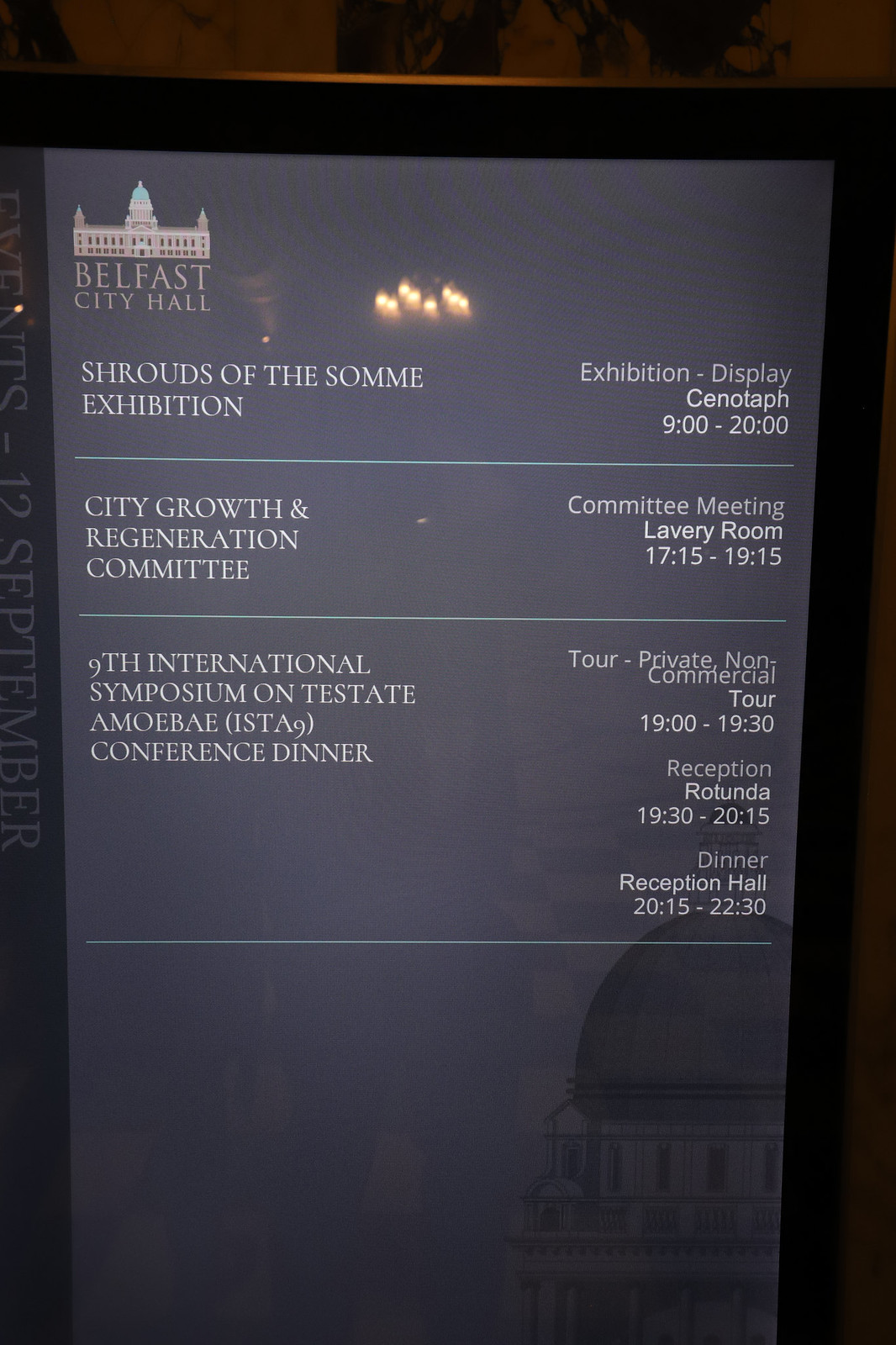The image is a tall, rectangular digital menu displayed against a dark gray background with white text, bordered by a thick black frame. At the top left corner, there is a light pinkish-beige text that reads "Belfast City Hall," accompanied by a digital illustration of a grand two-story building with a central column topped by a turquoise dome. This image provides information on various events happening at Belfast City Hall. The first event listed, in white font, is the "Shrouds of the Psalmist Exhibition," taking place at the Cenotaph from 9:00 to 20:00. This is followed by the "City Growth and Regeneration Committee" meeting in the Lavery Room from 17:15 to 19:15. The final event is the "Ninth International Symposium on Testate Amoebae (ISTA-9) Conference Dinner" scheduled from 19:00 to 19:30. Each event description is separated by a green line, giving a structured and organized look to the digital menu.